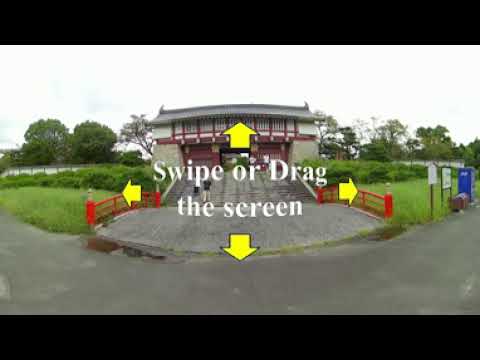The image depicts an outdoor interactive scene centered on a traditional Japanese temple with distinctive red and white architecture, including a pagoda-style roof and red gates leading up to it. Prominently displayed in the middle of the image are bold, yellow arrows pointing in all directions with the text "swipe or drag the screen," indicating that users can engage with the image for a 360-degree view. The temple is accessed by cement stairs that widen into a cement balcony before descending onto a concrete or asphalt walkway. There are a few people walking up the steps, enhancing the sense of activity. Surrounding the walkway are green bushes, trees, and a patch of grass on either side of the temple entrance. In the background, large trees and a fence frame the scene, while a blue porta-potty and signage, potentially informational or advertising-related, are visible to the right. The sky appears white, making it unclear whether the day is cloudy or sunny.